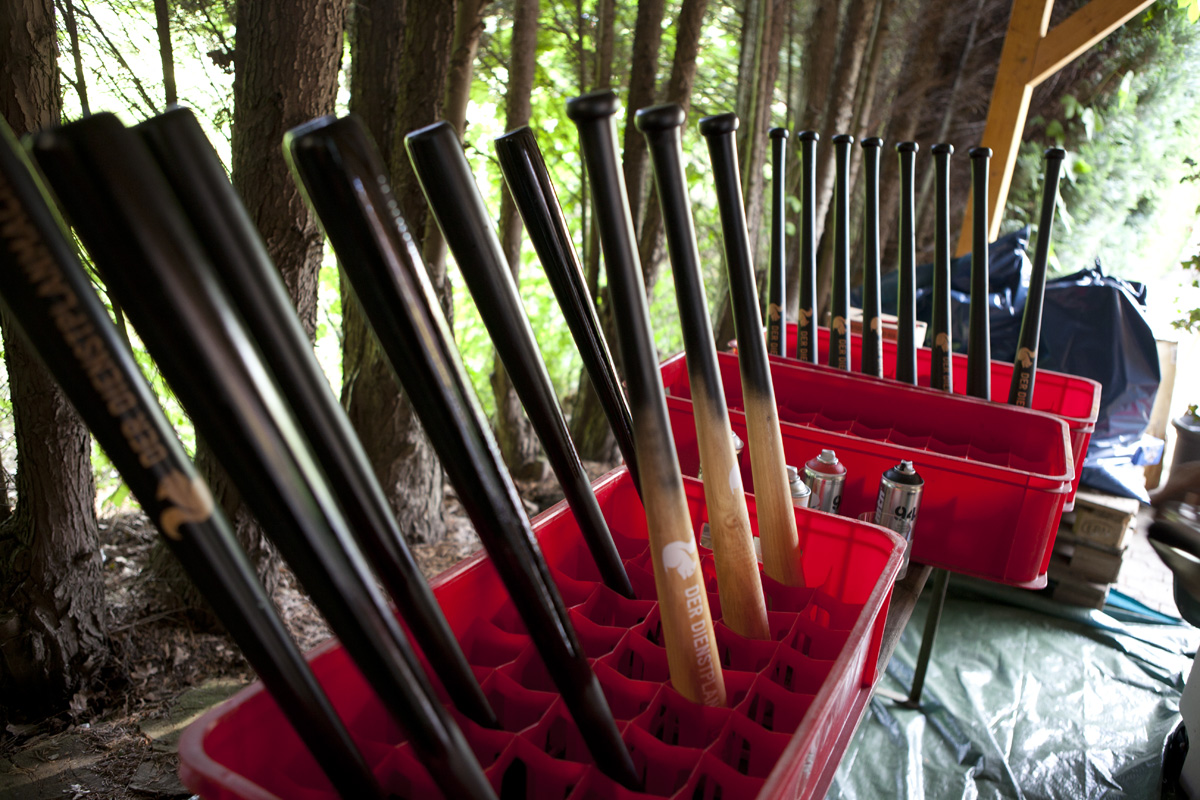Set against the backdrop of a sunlit forest with an abundance of trees, this photo showcases an intriguing scene of makeshift structures and scattered equipment. On the left, several trees tower amidst lush green vegetation, providing a natural setting. Central to the image is a collection of red plastic containers, prominently holding an assortment of baseball bats. The majority of the bats boast a sleek black finish, though a few are partially painted, revealing their original wooden grain. A green tarp lies underneath the containers, enhancing the outdoor feel.

Beside the containers, a mix of paint cans lies casually, hinting at ongoing customization work. Noticeable to the right is a blue bag, reflecting sunlight, while further to the left, a metallic object aligns with the scene. Supporting the containers are wooden boards and pallets, possibly forming the base of a rudimentary open-air shed-like structure. The sun's rays streaming through the leaves add a warm, natural illumination to the entire setting.